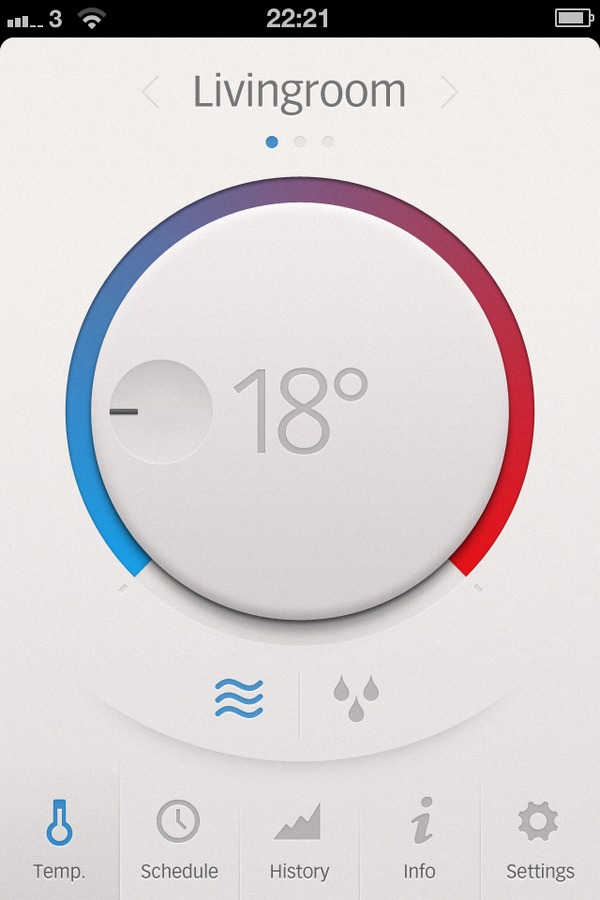A detailed description of the image:

The image depicts a smartphone screen displaying a thermostat app. At the top of the screen, typical status indicators are visible: three signal bars, the number '3', a partially-filled battery icon in a whitish-gray color, and the time, which reads 22:21.

Beneath these indicators, the word "Living Room" is displayed prominently in gray text, flanked by left and right arrows, suggesting the possibility to navigate between different rooms or zones.

Below the "Living Room" label, three small dots are visible, with the first dot highlighted in blue, indicating the current selection.

The central focus of the app is a large white circle showing the thermostat set to 18 degrees. Inside this larger circle, there is a smaller circle bisected horizontally by a line, which does not extend fully across and includes a tiny circle on the line. Encircling the thermostat setting are red and blue arcs that blend towards the middle into a light purplish hue, indicating a mix of heating and cooling options.

At the bottom of this main circle, three wavy blue lines can be seen, representing air flow or a fan, accompanied by three gray raindrop icons, likely denoting humidity or moisture settings.

Directly beneath the temperature display, several icons represent various app features: 
1. A temperature icon labeled "Temp".
2. A clock icon labeled "Schedule".
3. A mountain range icon labeled "History".
4. A lowercase “i” icon labeled "Info".
5. A star-shaped icon resembling a settings gear labeled "Settings".